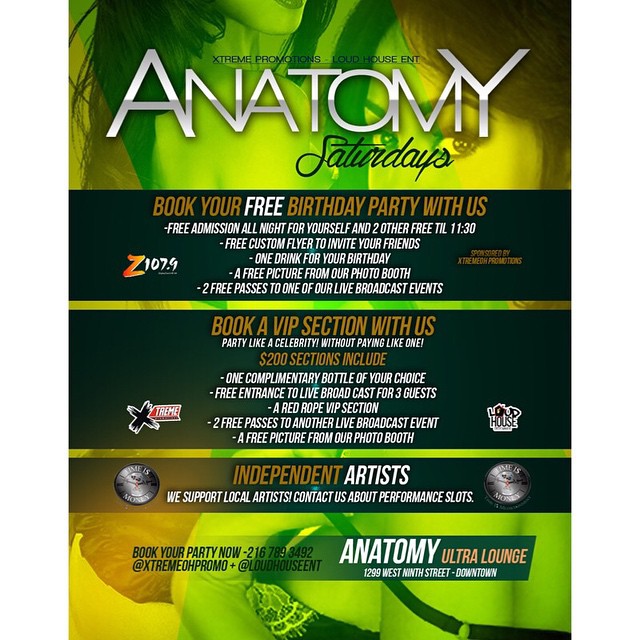This detailed vertical information card advertises events at Anatomy Ultra Lounge, primarily focusing on their Saturday promotions. The background features a gradient of green with a splash of orangey-yellow in one corner, accented by three black bands that convey essential details. At the top, in bold white letters, it reads "Anatomy" with "Saturdays" in black cursive underneath.

The first black band highlights an enticing offer: "Book your free birthday party with us." Below, in white text, it elaborates on the perks - free admission all night for the celebrant and two guests until 11:30 PM, a custom flyer, one complimentary drink for the birthday person, a free photo from the photo booth, and two passes to live events.

The second band encourages visitors to "Book a VIP section with us." Detailed benefits for a $200 VIP package include a complimentary bottle (likely champagne), entrance to a live broadcast with red rope VIP section, two additional passes to live events, and another complimentary photo booth picture. This section also features logos for Extreme Promotions and Loud House Entertainment, sponsors contributing to the overall enticement.

The bottom band emphasizes support for local independent artists, with "independent" standing out in gold text, whereas the rest of the text remains in white. It invites artists to inquire about performance slots and provides a contact number for booking parties.

The card prominently includes sponsorship by radio station 107.9, adding credibility and excitement to the events. The overall color scheme includes white, black, brown, red, and golden accents, complementing the green and yellow background. This well-crafted advertisement captures the vibrant, supportive, and festive atmosphere of Anatomy Ultra Lounge on Saturdays.